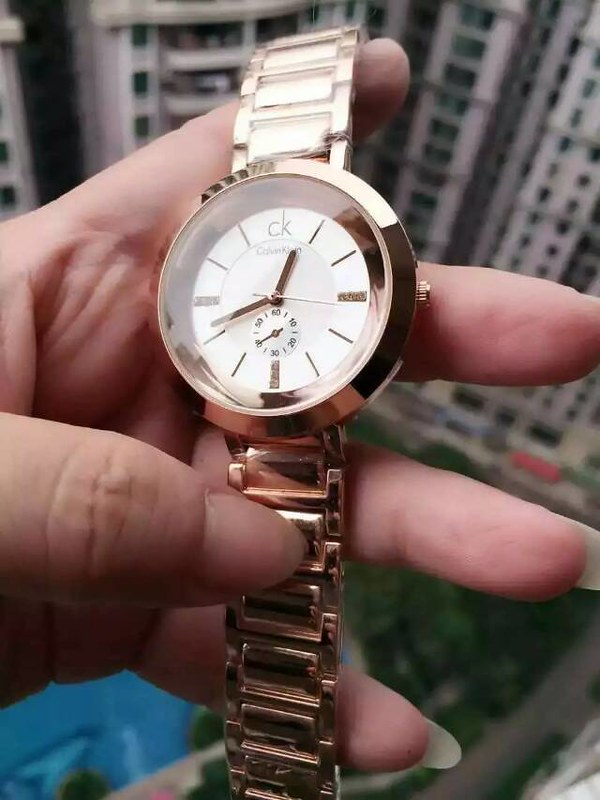The image captures a vertical rectangular photograph with a detailed foreground and a complex background. Dominating the center foreground is a left hand, presumably feminine, characterized by light-colored, thin fingers with long nails extending about half an inch from the tips. This hand, with the thumb and fingers spread to display the item, holds a watch by its metal band, revealing intricate details of the timepiece. The watch boasts a bronze-colored metal frame and wristband. Its face is white, marked with slender gold dashes in place of numbers, with slightly elongated bars at the 3, 6, and 9 positions, while the 12 is replaced by a small, bronze-colored "CK." Additional intricacies include a smaller inner circle marked from 10 to 16, aiding in precise time measurement.

The background reveals a bird’s-eye view, suggesting the photo might have been taken from a high vantage point, possibly a balcony or hotel window. The cityscape shows several tall, gray skyscrapers with black windows. Below, a blue pool with a tan border, green bushes, and trees lining a road with parked cars add perspective and depth. The image encapsulates a blend of urban architectural beauty and the elegance of a meticulously detailed timepiece in the foreground.